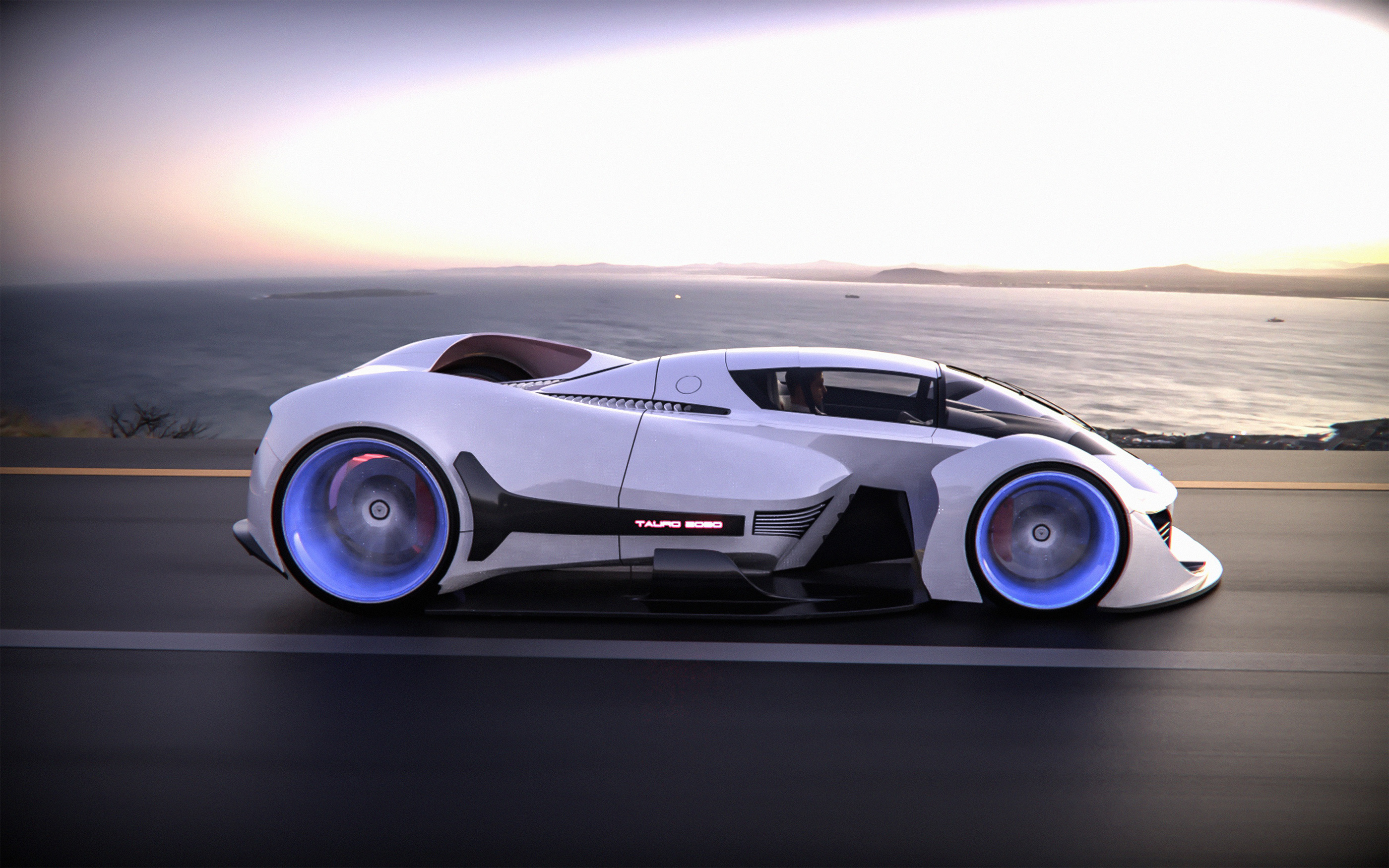This image showcases a sleek, futuristic concept car traveling from left to right on a gray asphalt road. The car features a pristine white body and eye-catching glowing blue wheels, with the front wheel smaller than the back one. It bears a distinct black line along its side, inscribed with "Toro 2030" in white text. The vehicle’s design highlights a rounded, dome-shaped windshield reminiscent of a jet fighter cockpit, and a low front scoop that enhances its aerodynamic profile. Sunlight bathes the scene with a warm yellow glow, which transitions into a bright white sky above. In the background, an ocean or lake stretches out, with gentle waves visible and an island faintly appearing on the horizon.